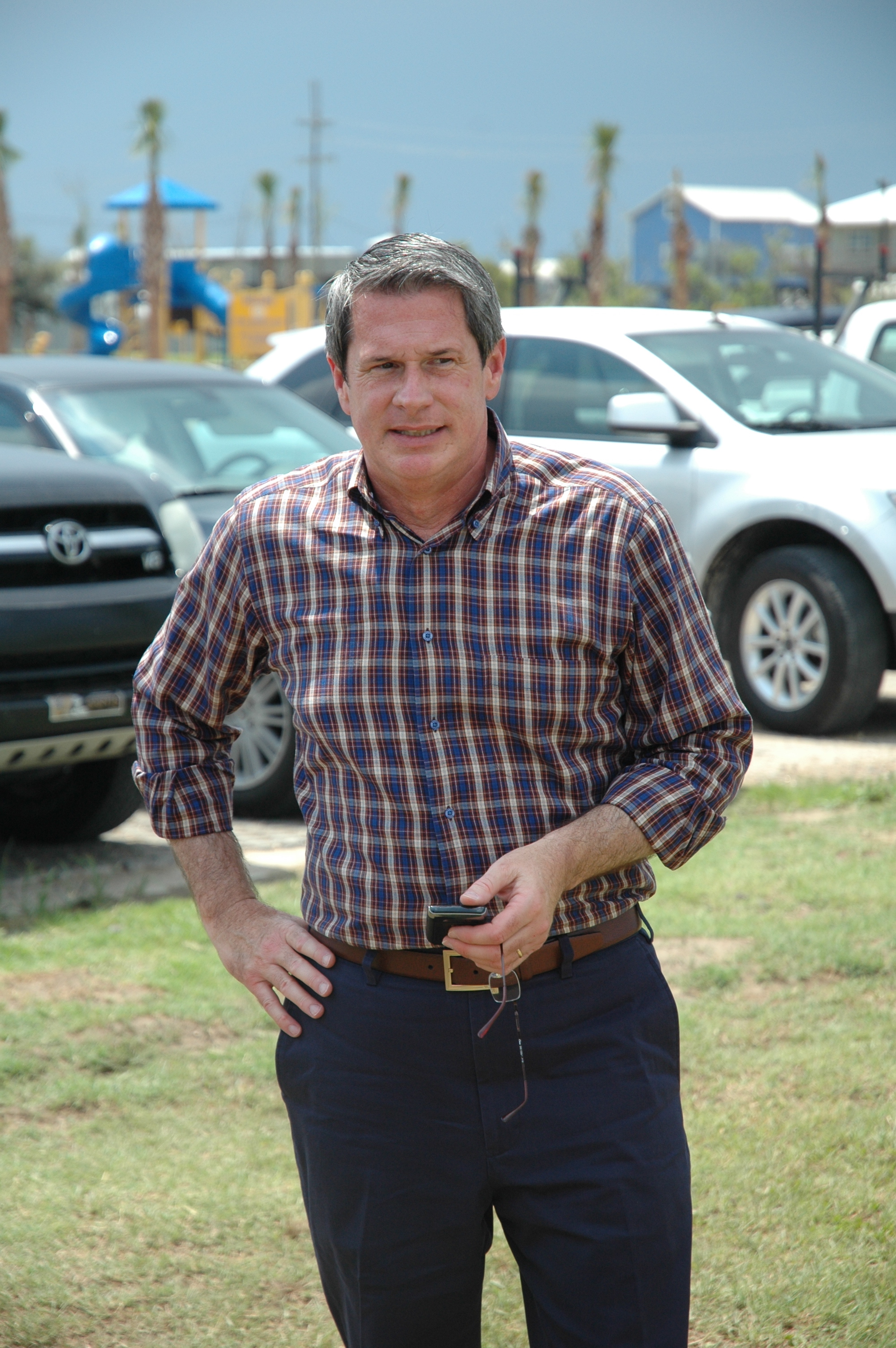The image features a man standing outside on a lush, green lawn, positioned directly in the center of a vertically oriented photo. He has short, straight gray and black hair combed to the side and is dressed in a tucked-in checkered flannel shirt with rolled-up sleeves, featuring a pattern of dark colors like reddish, blue, and brown. He wears a brown leather belt, dark navy chino pants, and is holding a pair of glasses intertwined with a cell phone in one hand, while his other hand rests on his hip, giving a slightly posed appearance. His subtle smile contrasts with a hint of a disappointed or upset expression. In the background, a row of parked cars—including a Mitsubishi, a white car with large tires, and an SUV with a Toyota symbol—can be seen. Further behind, there's a blur of colorful tents, umbrellas, and white-roofed structures with poles. Palm trees and a playground are visible in the distance beneath a light sky blue expanse.